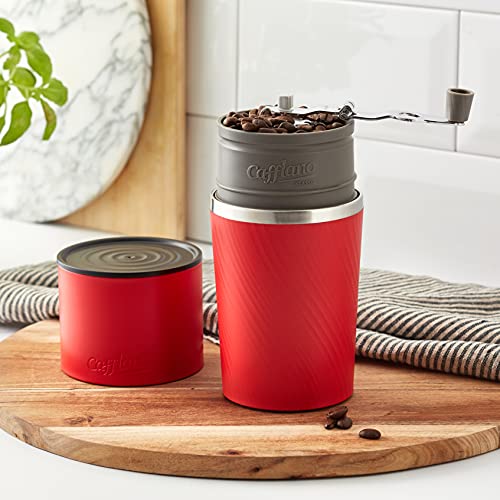The photograph showcases a detailed scene centering on a vibrant coffee grinder. The grinder, composed of a red cup at the bottom and a gray cylindrical middle, stands prominently on a circular wooden cutting board, which itself rests on a white kitchen cabinet. The detachable red lid of the grinder sits to the left, revealing the gray interior filled with roughly ground coffee. A handle is attached for manual grinding, allowing the user to rotate and crush the coffee beans. Scattered on the cutting board in front of the grinder are a few whole coffee beans. In the background, a hand towel with gray and brown stripes adds a touch of texture, and to the left of the frame, there is a wooden panel likely associated with the kitchen décor, complementing the white, shiny tiled wall.